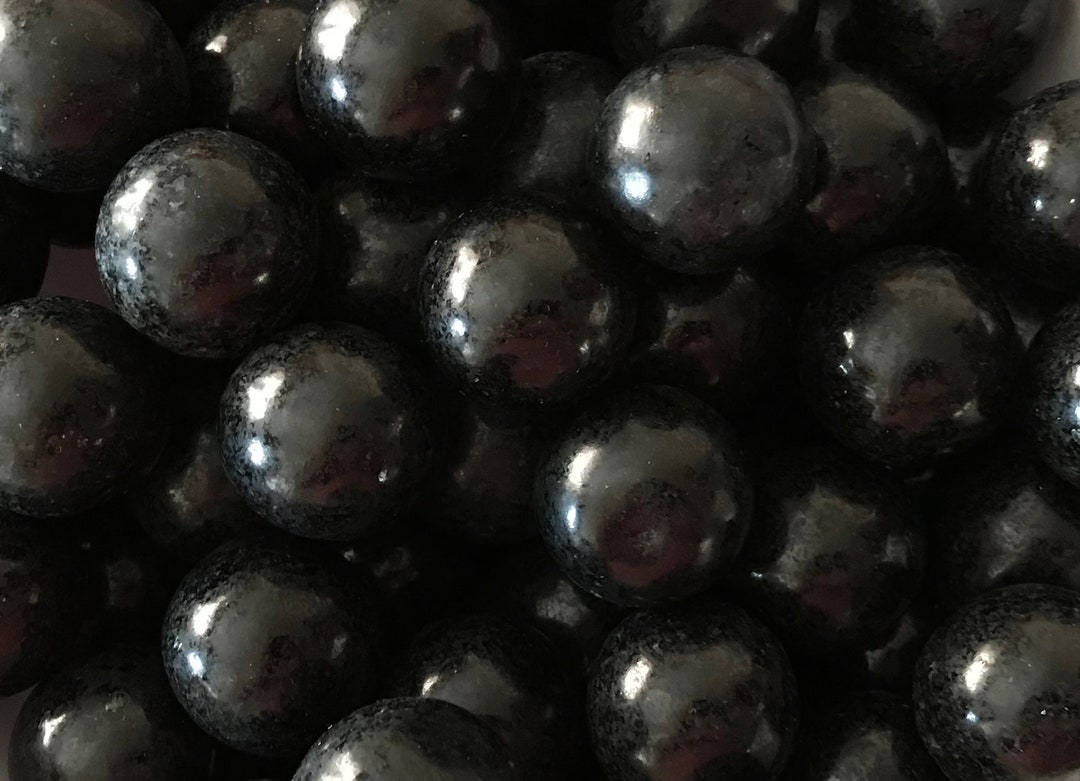In this rectangular photograph, we see a densely packed pile of small, round Java Plum fruits. The Java Plums, numbering in the dozens, are primarily black with a pinkish tinge on their tops. They are uniformly sized and shaped, appearing to be roughly spherical. The surface of some of these plums glistens, reflecting white light that creates small, shiny dots. The fruits are stacked closely together, filling the entire frame of the image. Despite some confusion about their exact nature, it is clear these are not marbles, gumballs, olives, nor grapes, but indeed glossy Java Plums captured in a highly detailed and reflective manner.